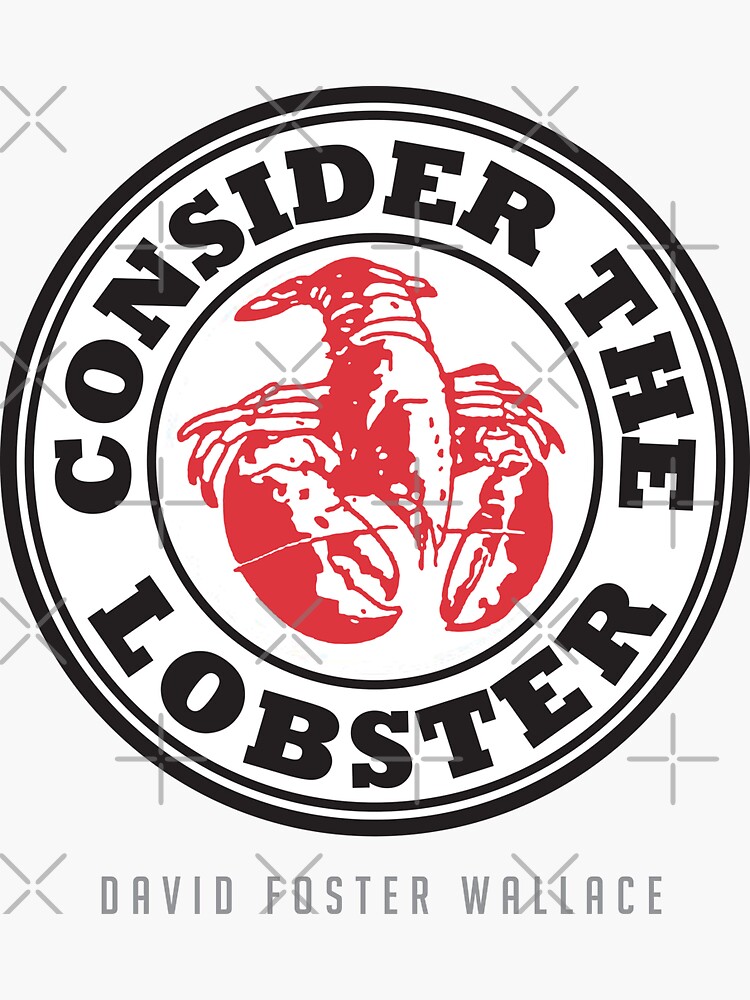The image is a graphically designed book cover featuring a light gray background adorned with scattered X's and plus signs. Central to the design are two concentric black circles. Between these circles, the words "CONSIDER THE LOBSTER" are inscribed in bold, black, capital letters. Inside the innermost circle is a detailed red lobster graphic, positioned with its tail and legs visible and its pinchers pointed downward. Below this image, the author’s name, David Foster Wallace, is written in capital letters in light gray text.